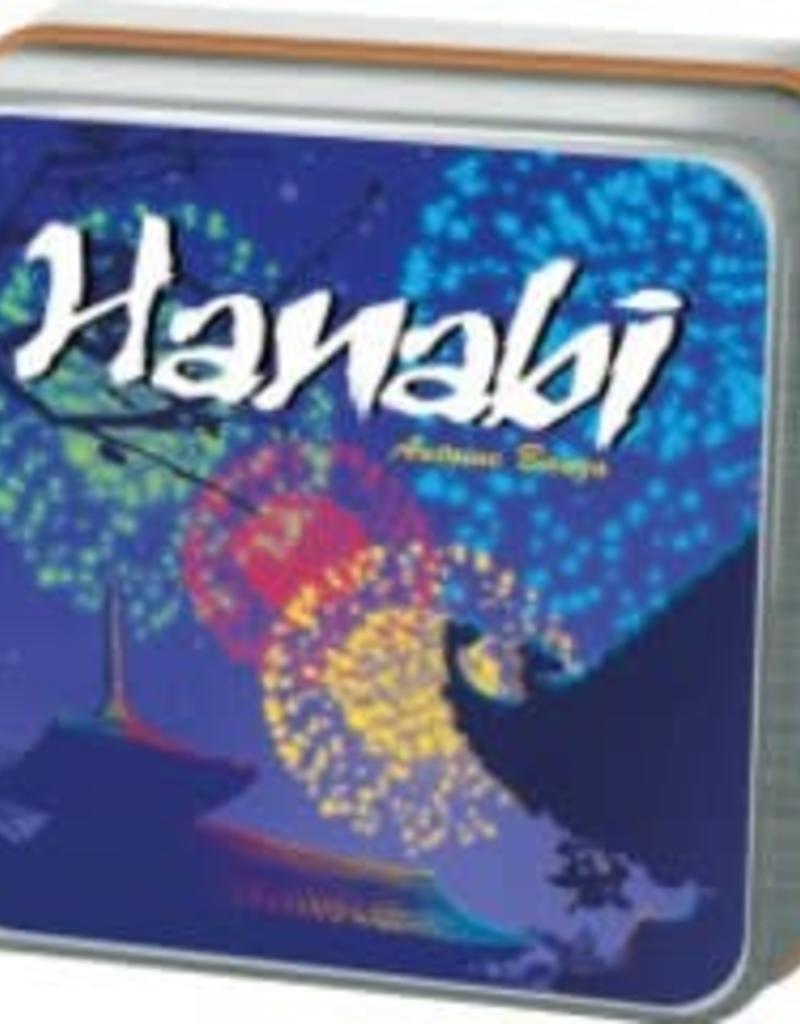The image appears to depict the front surface of an old metal container, possibly a lunchbox, taking up the entire frame. The container has a blue background that mimics a starry night sky and prominently features the word "Hanabi" in large white letters near the top. Directly below "Hanabi," there's some smaller, blurry yellow text that is unreadable. The central design includes several starburst, firework-like graphics in vivid colors: a large yellow one, a red one, a green one, and a blue one. These colorful bursts seem to overlap artistically across the container.

In the lower region of the container, on the left side, stands the image of a building reminiscent of a traditional pagoda, complete with a roof and a tall, pointy spire reaching towards the sky. Adjacent to this structure, there appears to be another dark roof, barely visible in the shadows. The metal container itself is outlined by a silver frame, with a strip of brown along the top edge, framing the blue starry sky and the fireworks. On the right side of the container, there is a dark shape, possibly resembling the silhouette of a witch's hat or another indiscernible object. Overall, the container's design conveys a festive night scene filled with vibrant firework displays and an intriguing architectural element.